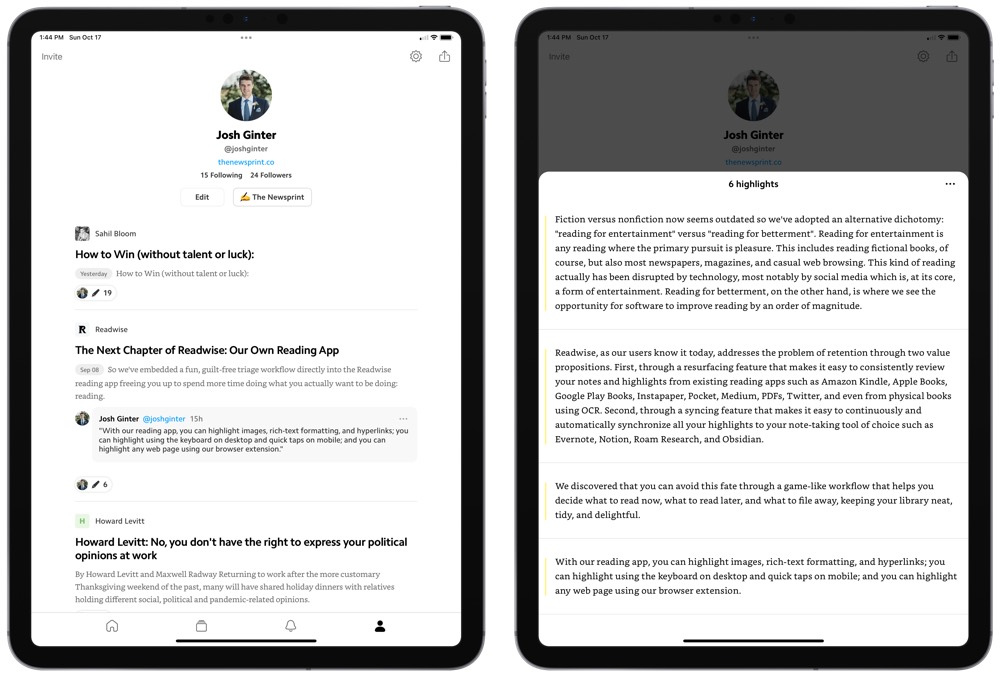In this image, we see two black-cased tablets displayed side by side, each in a vertical orientation. The devices are set against a sleek black background, emphasizing their modern, minimalist design. 

The tablet on the left features a social media profile with a white background. At the top, there is a profile picture of a young man, followed by the name "Josh Ginter" in bold black text. His username, "@JoshGinter," is displayed beneath the name, alongside follower statistics showing 15 following and 34 followers. Two buttons are visible: "Edit" on the left and a newsprint icon on the right. Below these, there are articles with titles such as "How to Win (Without Talent or Luck)" and "The Next Chapter of ReadWise, Our Own Reading App." Small, indeterminate icons appear beneath these titles, although they are somewhat blurry and hard to identify.

The right-hand tablet partially overlays the left one, and across its screen, a window with text is visible. The top of this overlay reads, "6 Highlights," followed by four discernible paragraphs of text, indicating a focus on detailed content or possibly an e-reader feature.

Overall, the scene captures a moment of digital interaction, emphasizing the sleek design of the tablets and the depth of content accessible through them.